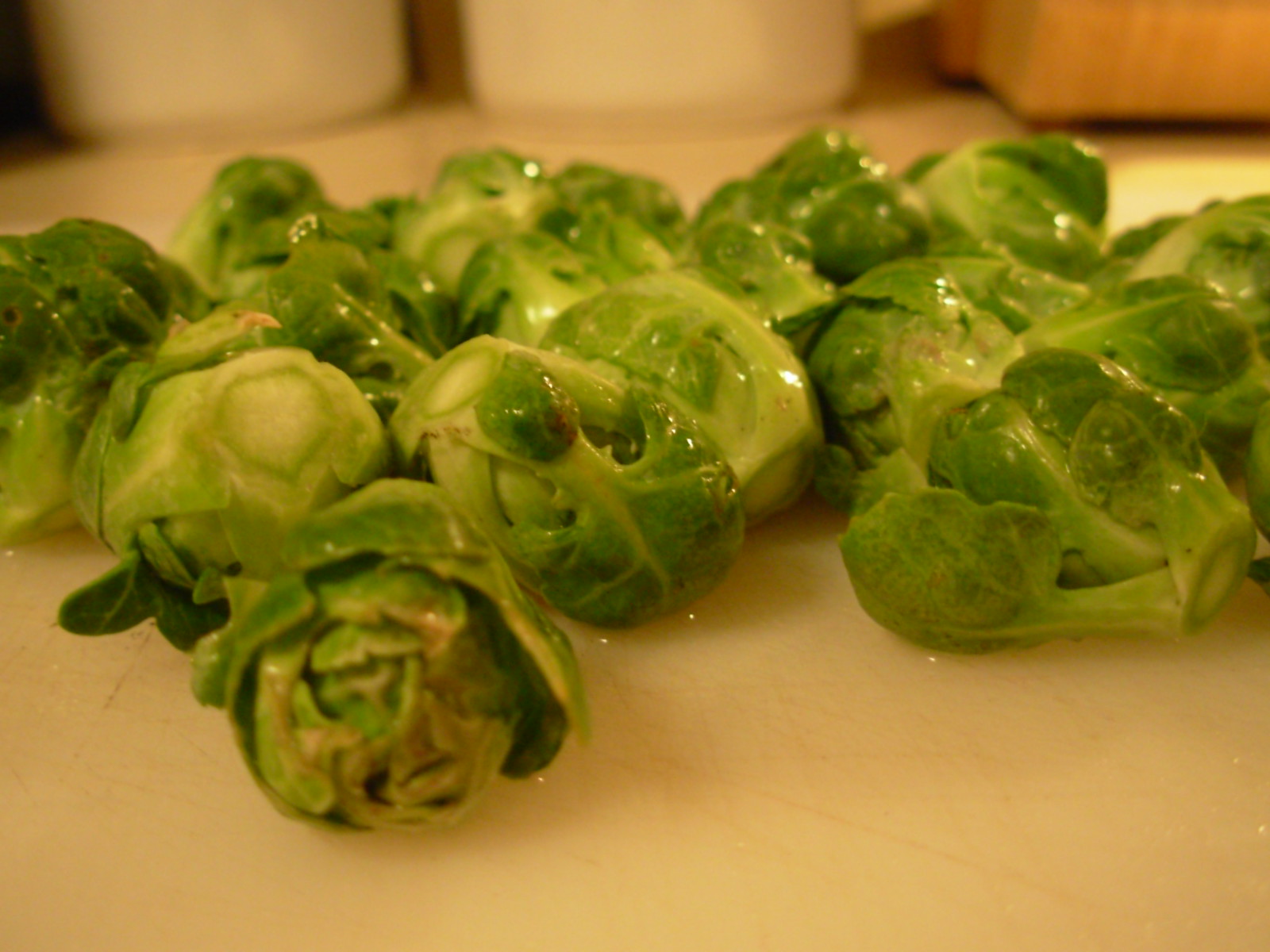This photograph captures a close-up of approximately a dozen freshly washed brussel sprouts, glistening with water droplets. The sprouts, small and circular, exhibit a bright green hue with a few displaying subtle brown patches, possibly due to sun exposure. They rest on a white cutting board, evident by the pooling water and visible knife marks. The brussel sprouts have cleanly cut bottoms and are neatly arranged on the board, which is situated on an off-white kitchen counter. In the blurred background, there are hints of white porcelain jars and a wooden block, anchoring the scene in a kitchen setting.